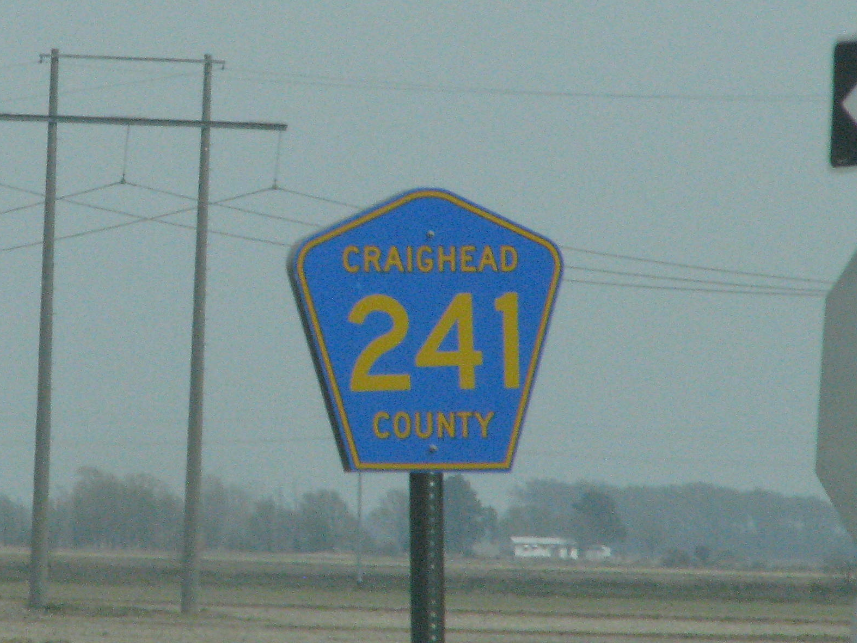The rectangular image, oriented horizontally, prominently features a road sign at its center. The sign is pentagonal, with a blue face and a yellowish-orange border. Bold yellowish-orange text in the middle reads, "Craighead County 241." The sign is mounted securely on a post, attached by two bolts, one at the top and one at the bottom.

In the background to the left, a tall electrical pole with multiple wires extending both to and from it adds depth and context to the scene. The sky is overcast, filled with thick clouds. Below the sign, the landscape includes trees, a distant house, and open fields, providing a contrasting natural element to the constructed elements of the photograph.